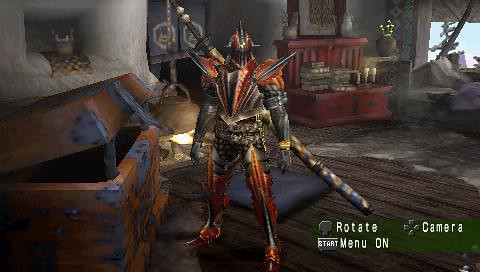This is a screenshot from a video game set in a detailed 3D environment, focusing on a heavily armored, imposing warrior. The character stands out due to his broad shoulders and dark, slate-gray armor adorned with red and gold highlights. His face is completely obscured by an elaborate helmet that features blade-like protrusions on the crest and shoulders. Strapped to his back is an enormous katana, matching the dark gray and gold color scheme, with floral and blue splotches adorning the bottom of the blade.

Surrounding the warrior is a richly detailed room, possibly an attic, with various pieces of furniture and loot. To the left of the character is a large, empty treasure chest made of redwood with metal reinforcements and a steel lock. Behind the chest, there's an alcove containing a pot with glowing mushrooms sitting on a checkered cloth. Adjacent to this is a piece of furniture resembling a hutch or dresser, filled with books, white candlesticks, and vases. The room features flagstone flooring and a brown and black striped rug.

On the right side of the image, an open window reveals a blue sky and the top of an evergreen tree, suggesting the room is part of a stone building, as indicated by the stone walls around the window. The game interface elements are visible in the foreground, including a green rectangle with instructions for rotating the camera, opening the menu, and navigation controls. Overall, the scene combines a medieval fantasy ambiance with intricate details to enhance its visual storytelling.